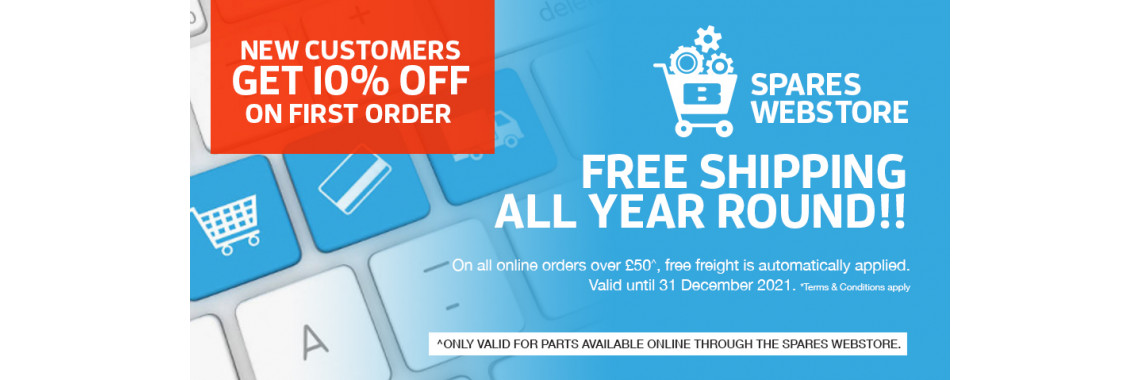**Caption:**

This advertisement highlights a special promotion for new customers at Spares Webstore, prominently displayed in a vibrant red banner on the top corner. The banner announces, "New Customers Get 10% Off on First Order," with the discount text emphasized in larger letters. The background features a sleek keyboard, giving a modern, tech-savvy feel. Below the banner, there are three blue buttons, each symbolizing different services: one with a shopping cart and credit card, another possibly representing delivery (a car icon), and a final button with an "A".

In the foreground, there's an image of a shopping cart filled with various objects, accompanied by a bold statement: "Free shipping all year round on all online orders over 50 pounds!" This offer includes a caveat that free freight is automatically applied and is valid until 31 December 2021, with terms and conditions applying.

Furthermore, a noticeable caret symbol highlights an exclusive detail: "ONLY valid for parts available online through the Spares Webstore." The overall advertisement positions Spares Webstore as a go-to source for spare parts, enticing customers with generous discounts and shipping benefits.